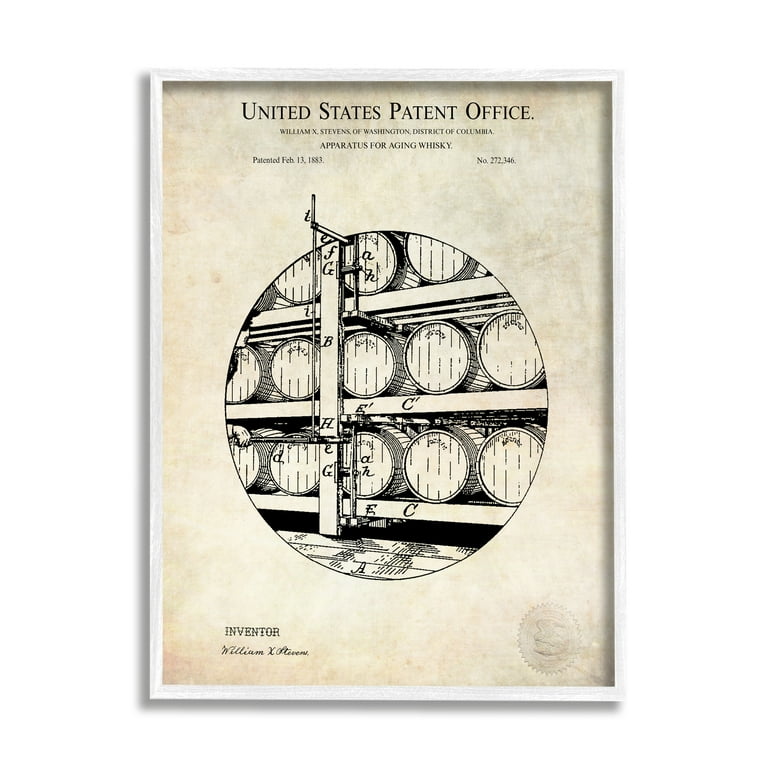This framed poster from the United States Patent Office, titled "Apparatus for Aging Whiskey," is a yellowed, cream-colored document dated February 13, 1883, and granted to William X. Stevens of Washington, D.C. The central feature is a large circle depicting an arrangement of wooden barrels on shelves, each marked with letters such as F, G, A, B, H, and C. The image is a stark, black-and-white sketch, typical of the period. The inventor’s name, William X. Stevens, is scripted at the bottom alongside the U.S. Patent Office seal. The poster, which also bears a distinct watermark, embodies the historical method of aging whiskey, reflecting the ingenuity of its time.